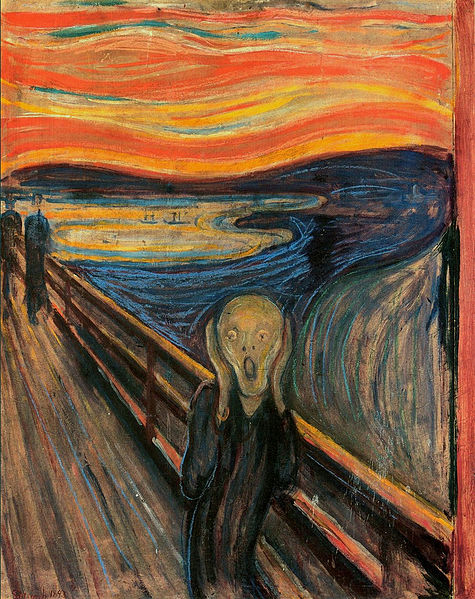The image showcases the famous painting titled "The Scream," often attributed to Edvard Munch. The artwork features a human-like figure with an elongated head and body, posed with its hands clasped against its cheeks, mouth wide open in a scream. The figure's form is slightly wavy, with a head almost resembling an upside-down pear shape. It is depicted with a bluish-green hue for the body and a pale face, standing on a pier with a wooden railing behind. The background includes two other figures walking along the pier, the deep blue water reflecting a hint of yellow from the setting sun, and a couple of small boats in the sea. The sky is vividly painted in impressionistic swirls of reds, oranges, and yellows with a touch of blue, suggesting a dramatic sunset. The shore is represented by a blend of tans and blues, completing this haunting and colorful scene.